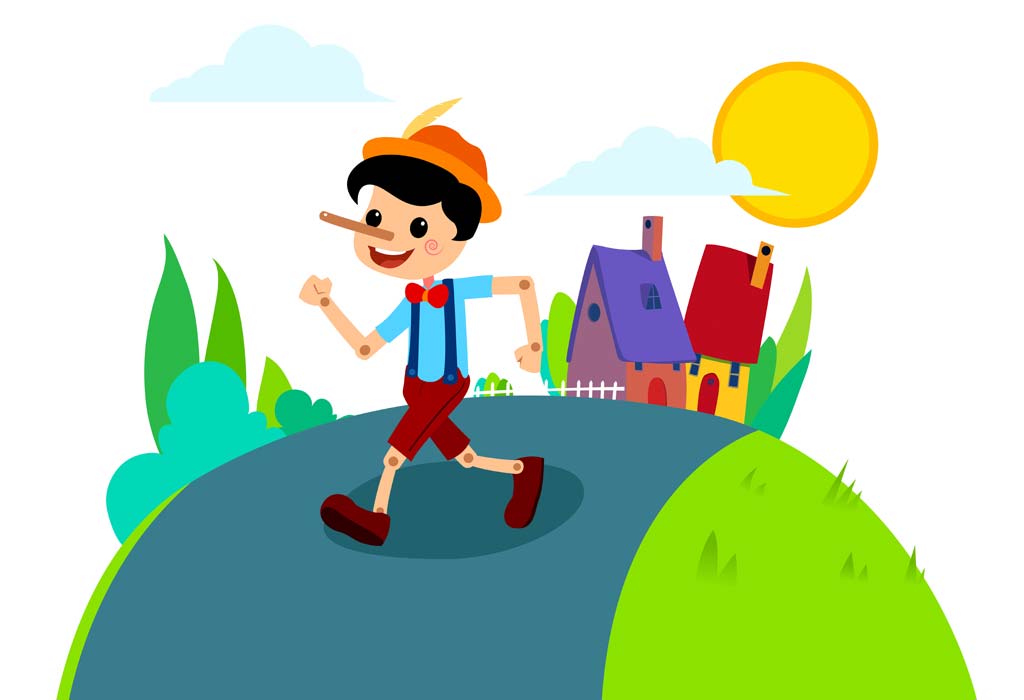This detailed image depicts a colorful, cartoonish scene featuring a Pinocchio-like figure. The character appears to be a young wooden boy wearing a short-sleeved blue shirt, orange bow tie, blue suspenders, brown shorts, and brown shoes. He has an orange hat adorned with a yellow feather, and his black hair peeks out from underneath. His most striking feature is his long, brown nose. Pinocchio is mid-stride with his arms bent as if he's power walking. 

In the background, the scene is bathed in a vibrant array of colors. There is a bright yellow sun with an orange border on the right-hand side of the white sky, which also features two light blue clouds with flat bottoms. The ground appears somewhat surreal, with a smooth, gray asphalt path winding through a landscape that includes light green grass dotted with darker green blades. To the left of the pathway, abstract trees and leaves in shades of green and blue create a whimsical woodland area.

Further in the background, there are two houses; one is orange with a purple roof and a chimney, while the other is yellow with a rust-colored roof and a chimney. This environment integrates plants growing around the houses, adding to the lush, animated outdoor scene. All these elements come together to create a vivid and joyful atmosphere, as Pinocchio strolls merrily along the pathway reminiscent of an enchanted, miniature world.